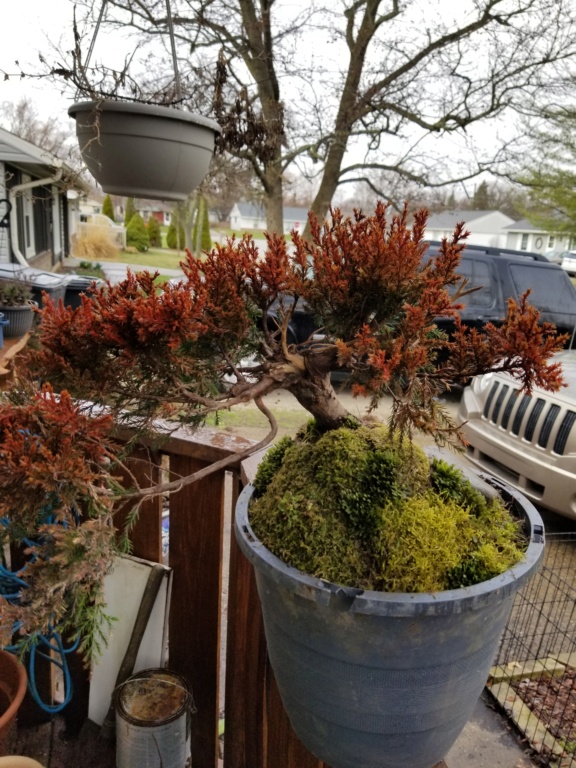In the center of the image is a potted plant with red leaves, resembling a bonsai tree, growing from moss-covered soil within a gray pot. This pot sits on a deck, possibly part of a front porch, and is surrounded by a stone driveway and walkway. Above the plant, a gray hanging basket is suspended from a deciduous tree in the front yard. The right edge of the image includes the grill and headlight of a silver Jeep SUV, with another larger black SUV visible parked nearby. In the distance, other houses of the neighborhood are visible under a daytime sky, creating a serene suburban outdoor setting.